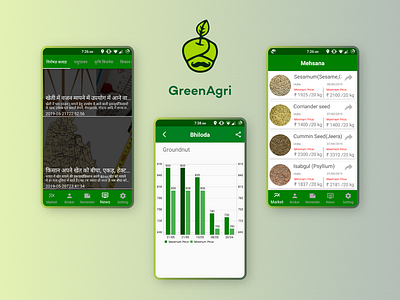The image features three phone screenshots surrounding a central logo and text. The logo, prominently displayed at the top center, depicts a stylized green turbaned man with a mustache and a leaf protruding from the turban, highlighted in light green and outlined in darker green or black. Beneath the logo, in green text, reads "Green Agri" with no spaces between the words. The phones show various screens related to the Green Agri app. The first phone screen, positioned on the left, displays a menu with several clickable items in white text, though specific details are unclear. The center screen shows a green bar graph, and the right-hand screen presents images of grains or small items, each accompanied by turned arrows, suggesting some interactivity or more information available. Overall, the arrangement and visuals emphasize the agricultural theme and functionality of the Green Agri application.